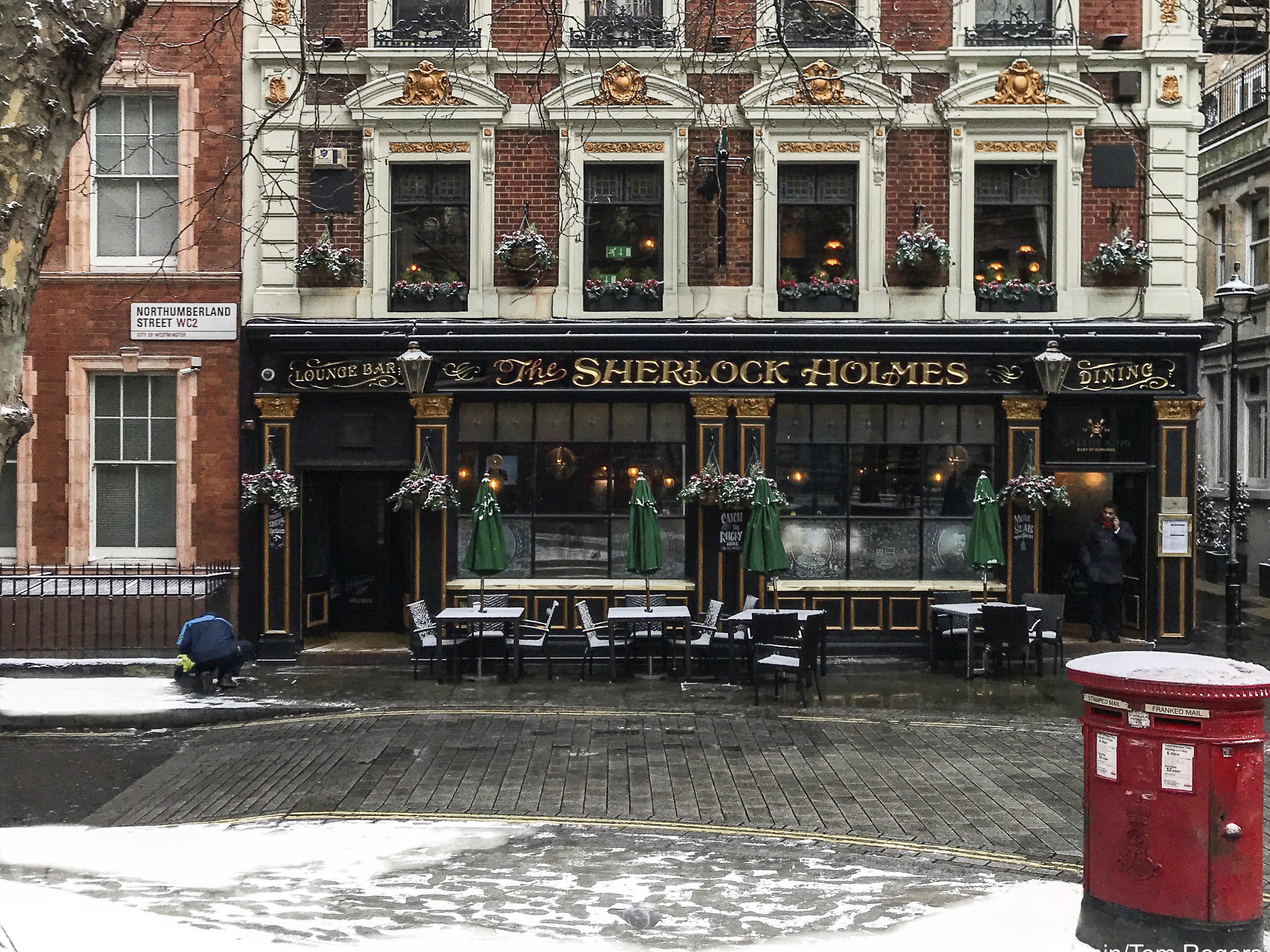The photograph captures a detailed, front-facing view of the Sherlock Holmes Dining and Lounge Bar, exuding a historical charm with its classic, architectural elements. The lower level of the building, painted entirely in black, features gold-trimmed columns flanking two prominent doorways positioned on the left and right sides, with large windows set between them. Above, a sizable sign in elegant gold lettering stretches across the façade, reading "Lounge Bar, The Sherlock Holmes Dining."

In front of the restaurant, there’s a quaint outdoor seating area with white tables and chairs, each adorned with green umbrellas that are currently folded inward. The scene is set on a gray brick street or sidewalk that runs along the front of the establishment.

The upper levels of the building showcase a red brick exterior accented with white-framed windows and gray stone detailing, including arched windows with gold trim. Flower boxes with blooming plants add a touch of color and vibrancy to the windows. The overall atmosphere suggests a cozy, yet refined dining experience inspired by the legendary detective Sherlock Holmes, all captured against the backdrop of neighboring red brick walls. The photo, taken during the daytime, emphasizes the building's historical appeal and the tranquil street setting.